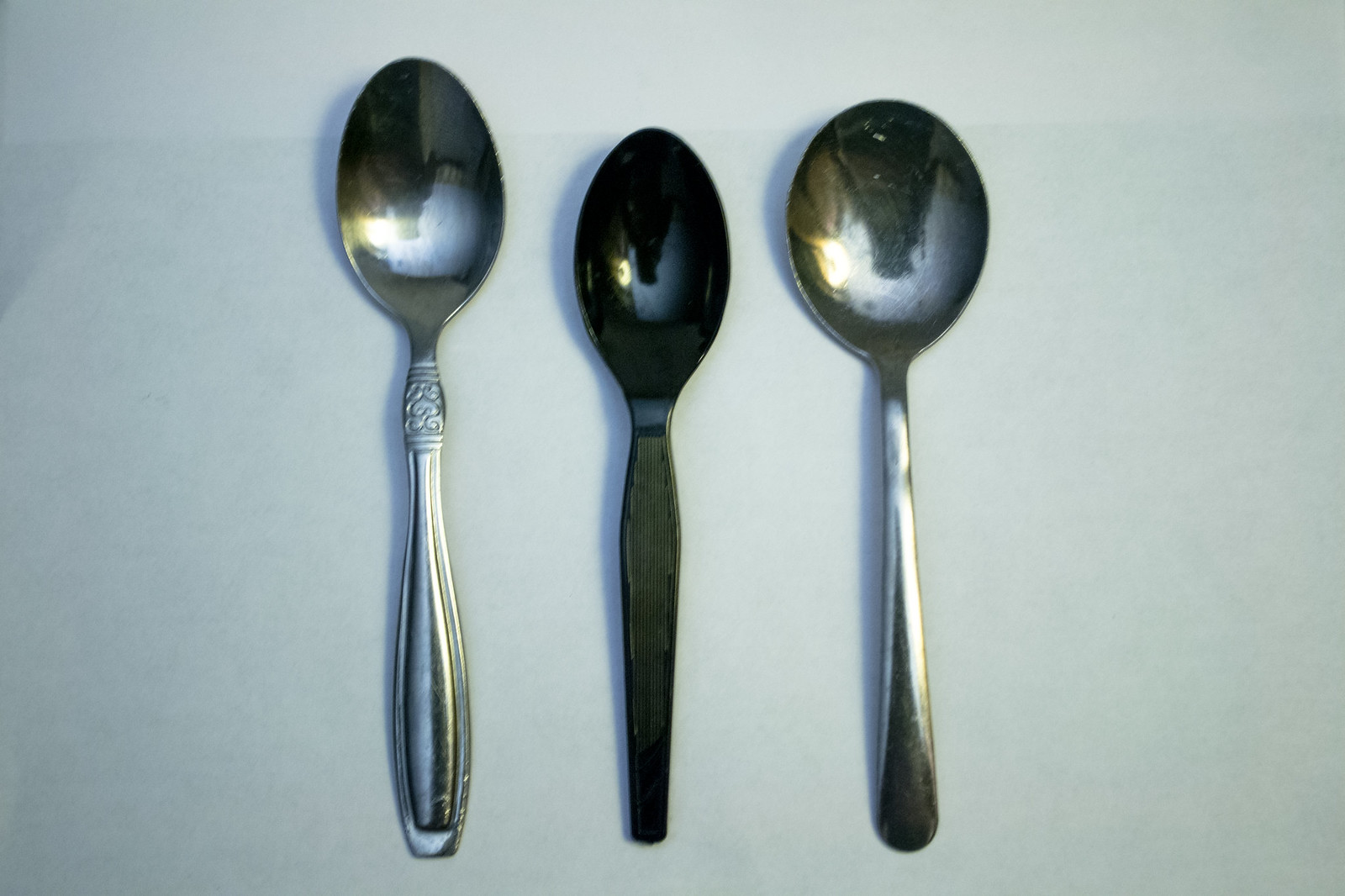The image captures three spoons resting on a very light surface, possibly a tablecloth or a piece of light-colored paper. The spoon on the left is the longest and is silver with an elegant oval bowl and an ornamental design where the handle begins. The middle spoon is notably smaller, appears black, and seems to be made of plastic or perhaps has a wood grain handle. The rightmost spoon is also silver, similar to the left spoon but it has a rounder bowl, characteristic of a soup spoon, and features a plain handle. Visible in the reflection on the spoons are the camera, photographer, and a lamp. The spoons have a slightly tarnished appearance, suggesting they could be antique.